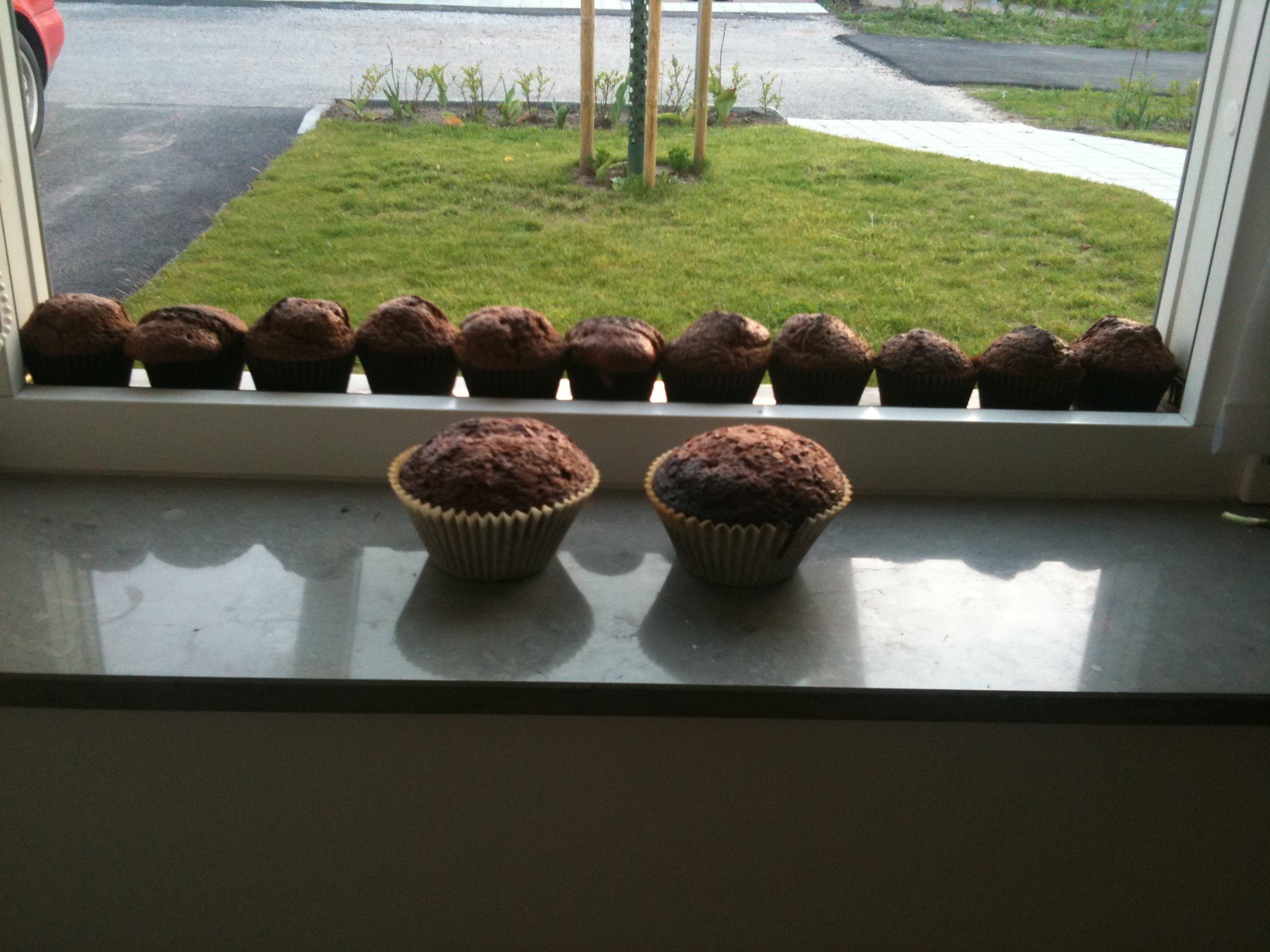In a cozy home kitchen, an inviting scene unfolds upon the windowsill and countertop. The windowsill, with its light grey ledge and white plastic inner frame, hosts a neat row of eleven chocolate muffins in dark brown cases. In the foreground, on the countertop, sit two slightly larger chocolate muffins, each nestled in white paper cases. The muffins are clearly chocolate and lack any icing, showcasing their rich, brown texture. Through the open window, a tableau of the outdoor surroundings is visible, featuring a lush, green patch of lawn, a stretch of black tarmac driveway on the right, and the red bumper of a parked car. To the left, the garden area reveals wooden posts supporting what could be a spiralized stake or perhaps the rough surface of a tree trunk, with green leaves and twigs sprouting at the curbside. The window offers a peaceful vista of the home's approach, lined with a grey concrete street and a path of white concrete leading to the entrance.